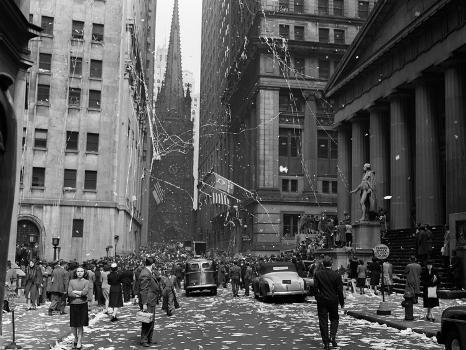This black-and-white photograph captures a bustling ticker-tape parade in downtown New York City, likely from the 1940s. The street is teeming with hundreds of people, overflowing from the sidewalks onto the asphalt below. Confetti and streamers rain down from high-rise buildings on either side, creating a celebratory atmosphere. On the right side of the foreground, there is a stately building with grand Greek columns and a triangular pediment, possibly a courthouse or government building, guarded by a statue that could represent a historical figure like Thomas Jefferson or Christopher Columbus. American flags are prominently displayed on the buildings lining the street, and paper debris is scattered everywhere. Among the crowd, a few vehicles, including an old delivery truck and a small coupe, navigate through the dense assembly. The street extends towards an intersection marked by a towering church steeple in the background, further emphasizing the grandeur of the scene and the historical significance of this exuberant celebration.